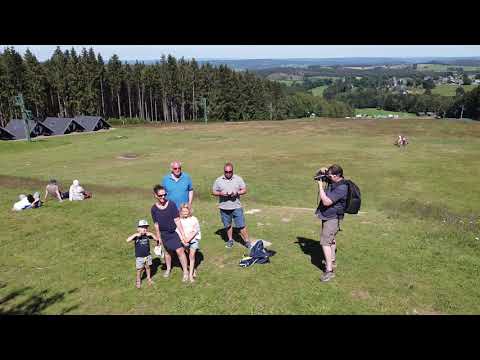In the image, a family of six is gathered in a vast, open field, bordered by trees on either side, defining the long rectangular plot of land. Central to the scene is a woman in a black dress and sunglasses, holding two children: a little blonde girl and a boy wearing a hat. Behind her stand two men; one is in a blue polo, and the other is bald, donning sunglasses, a gray shirt, and blue shorts. Next to them on the right, a man dressed in all black is capturing the moment with his camera. Additionally, there are three people sitting in the grass to the left, with three distant rooftops visible in the horizon. The lush green field and clear skies indicate it’s an outdoor setting in the middle of the day. The image captures a harmonious blend of family bonding amidst nature’s serenity.